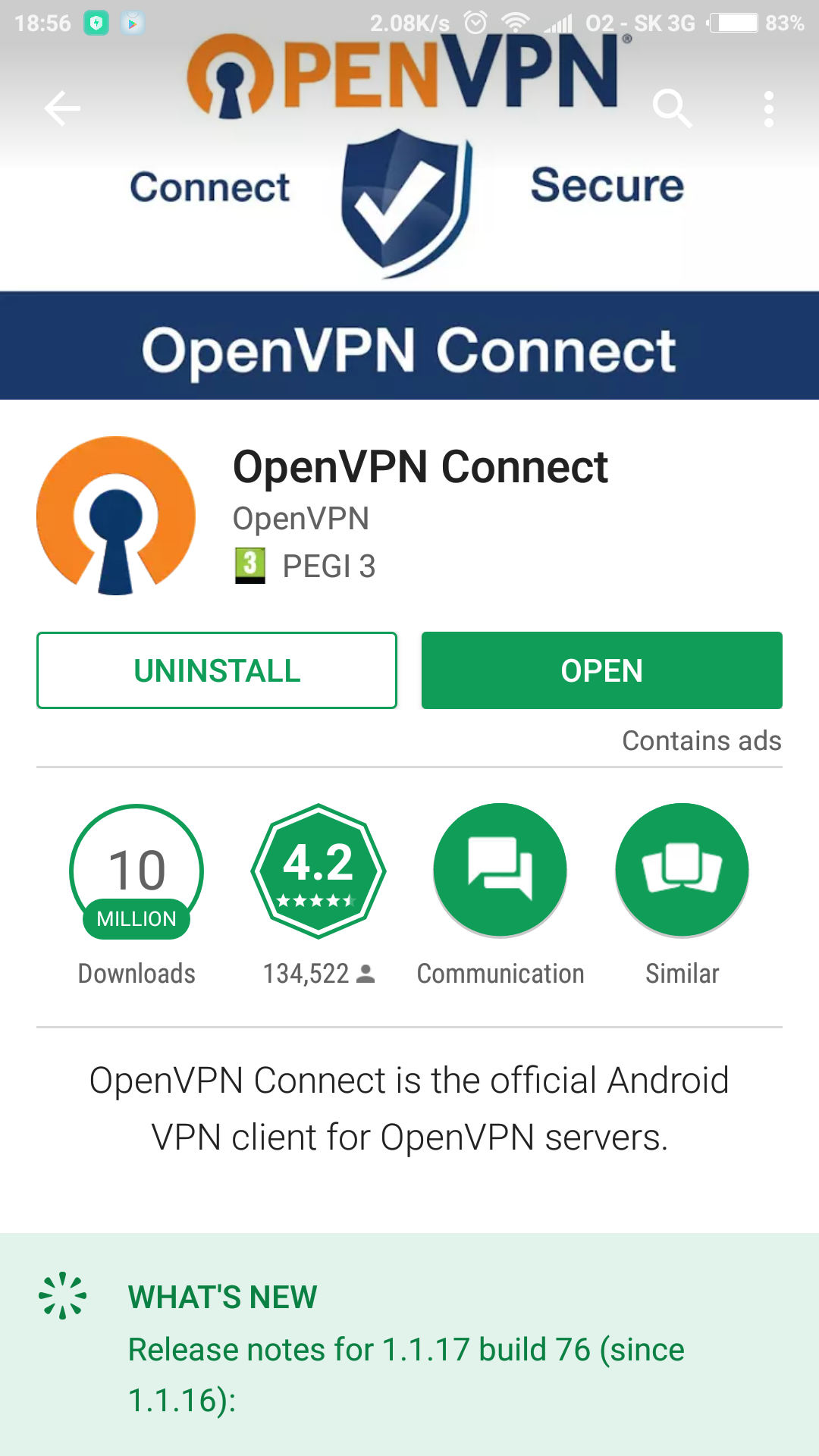This detailed image shows a screenshot of the OpenVPN app page on the Google Play Store. At the top center of the web page, the OpenVPN logo is prominently displayed. The word "Open" is depicted in orange letters with a small door lock icon replacing the 'O,' followed by "VPN" in blue letters.

At the very top of the screenshot, typical indicators from a cell phone are visible: the time on the left reads 18:56 (6:56 PM), and on the right, the battery status shows 83%. 

Directly below the OpenVPN logo, there is a tagline saying "Connect Secure," with a check mark and a small badge placed between the words "Connect" and "Secure." 

A blue bar follows, centrally displaying "OpenVPN Connect." Under this bar, the OpenVPN logo is repeated with "OpenVPN Connect" written next to it and is labeled "OpenVPN 3 PEGI 3."

The page features two prominent buttons: a white button with green text labeled "Uninstall" on the left and a green button with white text labeled "Open" on the right.

Below these buttons, four badges are arranged horizontally, providing key app information:
1. "10 million downloads"
2. A rating badge showing "4.2 out of 5 stars" based on "134,522 reviews"
3. A 'Communication' badge
4. A 'Similar' badge

Further down, a message reads, "OpenVPN Connect is the official Android VPN client for OpenVPN users," followed by the app's release notes.